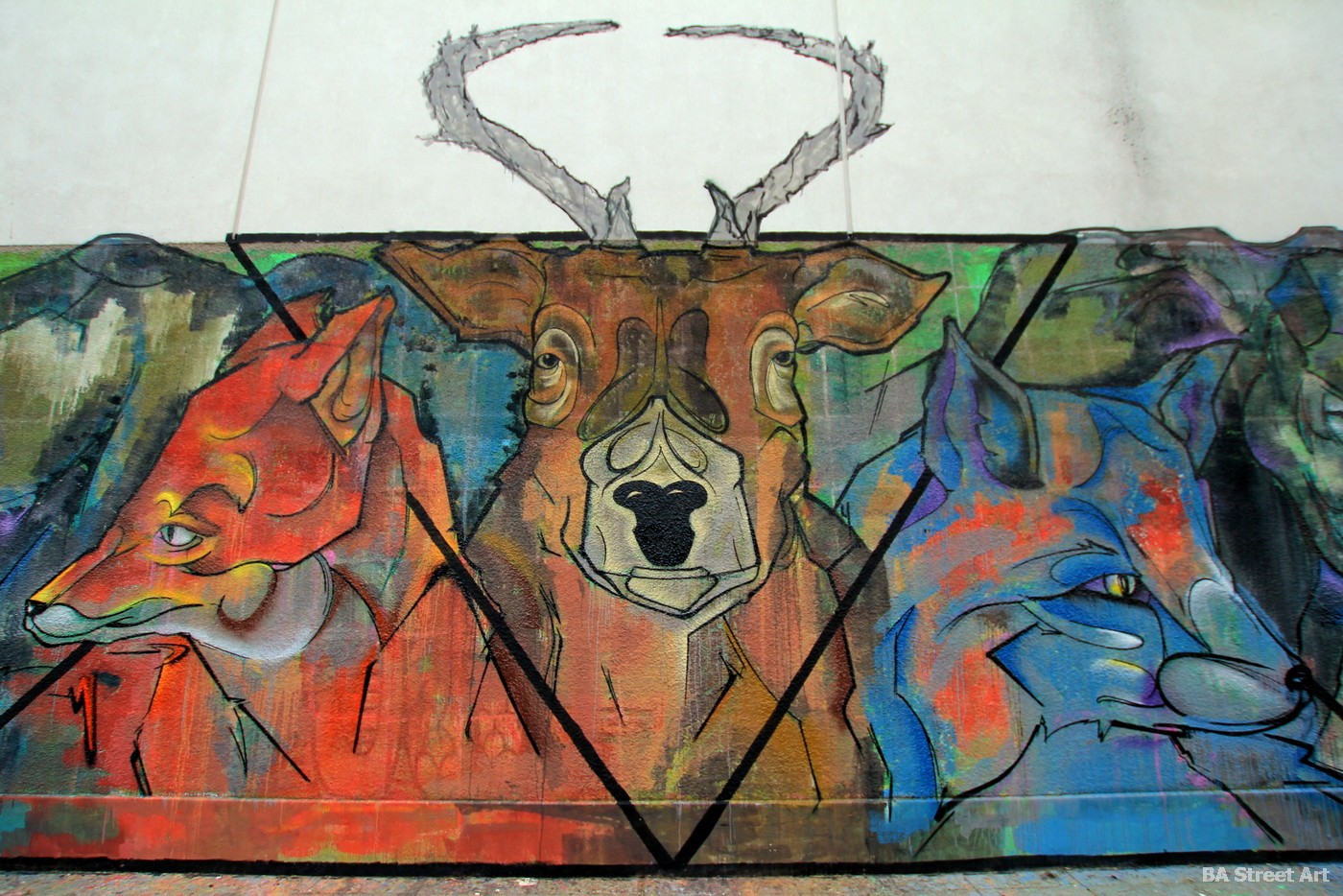The image features a large, vividly colored mural, likely painted with a brush rather than spray paint, depicting three distinct animals set against a predominantly white background. At the center of the composition is a majestic deer or elk, its chestnut-brown body facing forward. The deer’s antlers extend upward, breaking the colorful section and reaching into the white space above. Encircling the deer is a black-border forming an upside-down triangle. To the left side of the mural stands a reddish-orange wolf, its body oriented towards the viewer but with its head turned left towards the 9 o'clock position. On the right side, there is a blue fox with orange accents on its nose and cheek, its body also facing forward while its head looks right towards the 3 o'clock position. At the bottom right corner of the mural, the text "BA Street Art" is inscribed.